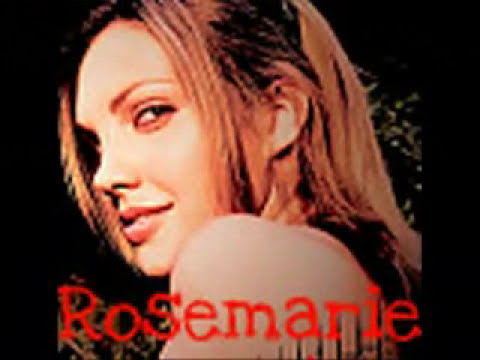The image appears to be reminiscent of old album artwork or a vintage CD case, featuring an up-close, side profile photograph of a young Caucasian woman with her head positioned at the very center and her left shoulder covering the bottom center. She has shoulder-length, brunette hair styled away from her face, with a few strands framing her features. She is dressed in a black tank top, exposing her left shoulder, and looking flirtatiously over her shoulder towards the viewer, showcasing a friendly, almost flirtatious smile. Her left eye is visible, while her right is obscured, and she sports thin eyebrows, a pointy nose, and full lips adorned with red lipstick. The backdrop is completely black, creating a stark contrast. At the bottom of the image, the name "Rosemarie" is prominently displayed in a large, red font, accentuating the minimalistic yet striking design. The overall image has a slightly blurry and pixelated quality, adding a nostalgic, old-school feel.